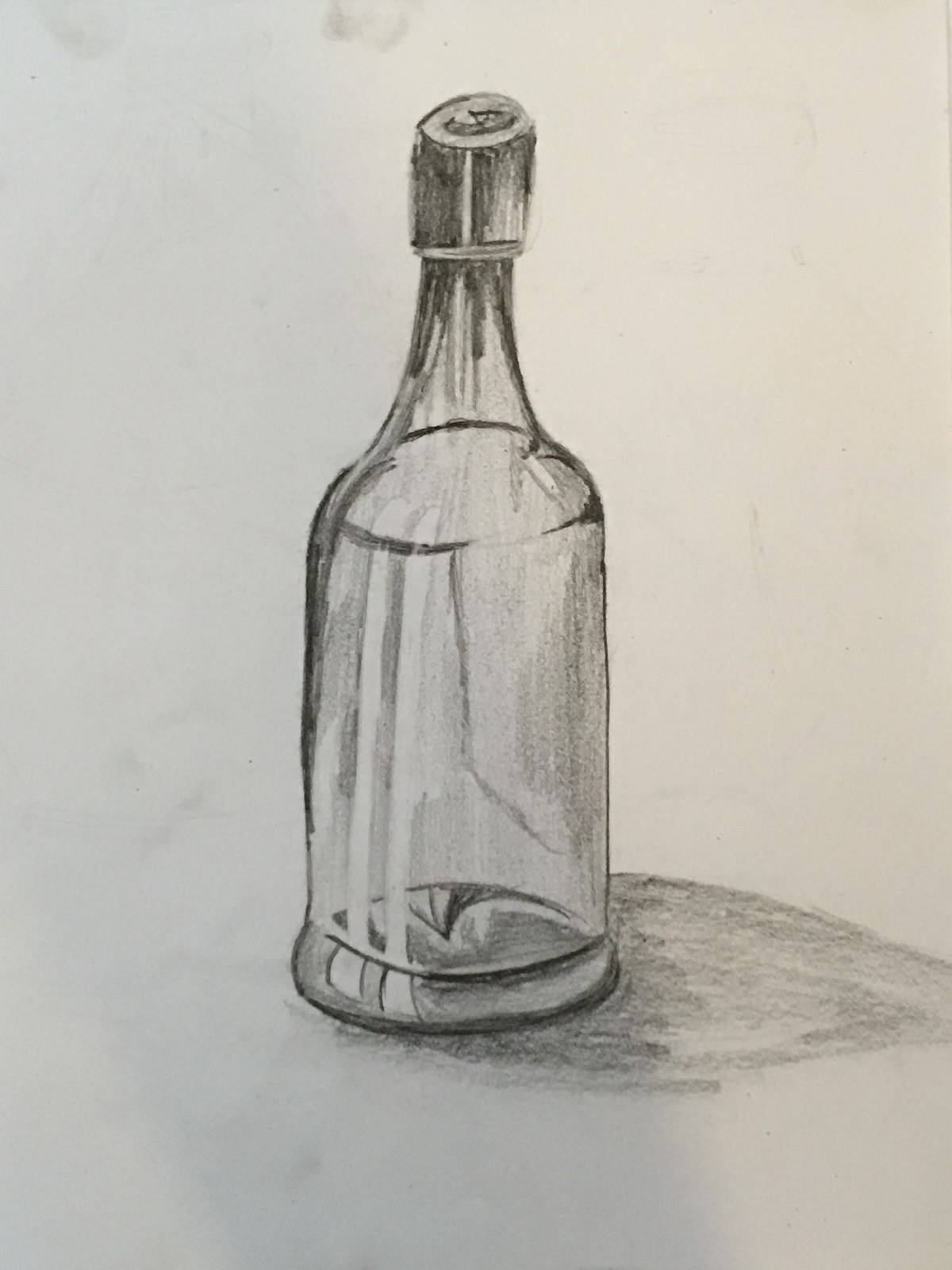This image features a detailed black and white sketch of a glass bottle on an off-white sheet of paper, slightly taller than it is wide. The bottle, reminiscent of a wine or booze bottle, has a wider cylindrical base that transitions into a curving neck, leading to a top covered by a plastic fitting. The fitting is slightly larger than the bottle's mouth and is marked with a 'C'. The sketch, likely done in pencil or charcoal, includes several smudges at the top left, possibly from the artist’s fingers. The bottle, which appears empty, shows two elongated white rectangles along its left side, possibly suggesting reflections or highlights. Additionally, a shadow-like form of the bottle is evident on the bottom right corner of the image. Various marks around the drawing enhance its textured, lifelike appearance.